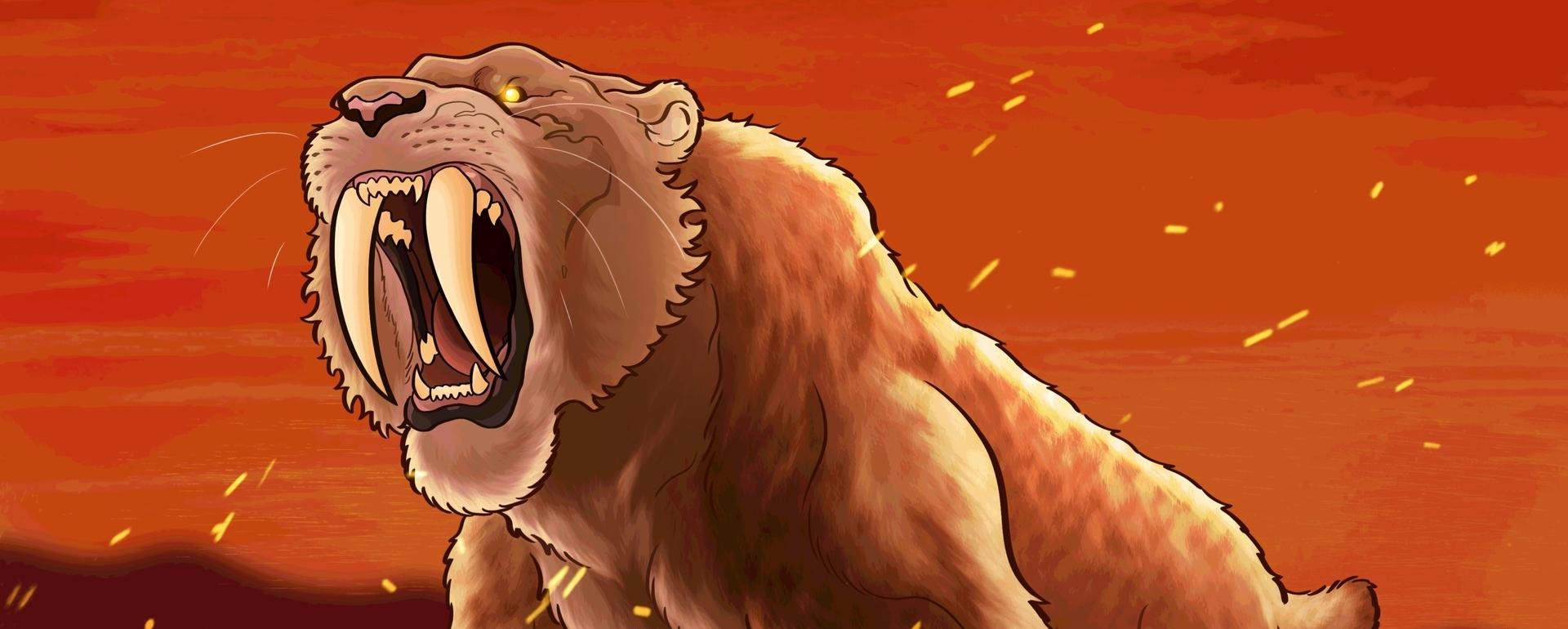This image appears to be a hand-drawn or animated still featuring a menacing saber-toothed tiger. The background is a vivid blend of deep red, orange, and yellow, reminiscent of a sunset or engulfed by flames, with streaks and tiny flares giving an impression of a fiery, dramatic scene. The saber-toothed tiger is shown in a close-up, prowling on all fours with a powerful and muscular build, featuring a brown coat with an orange glow. Its face commands attention with small ears, a black nose touched with purple, and fur outlining its face, which includes a noticeable mane. The tiger's mouth is wide open in a ferocious roar, displaying sharp lower teeth and enormous saber-like fangs that extend down dramatically. The detail in its yellow eyes and overall face adds to its intense and dangerous appearance. The short tail is visible towards the bottom of the picture, adding to the foreboding presence of the beast.